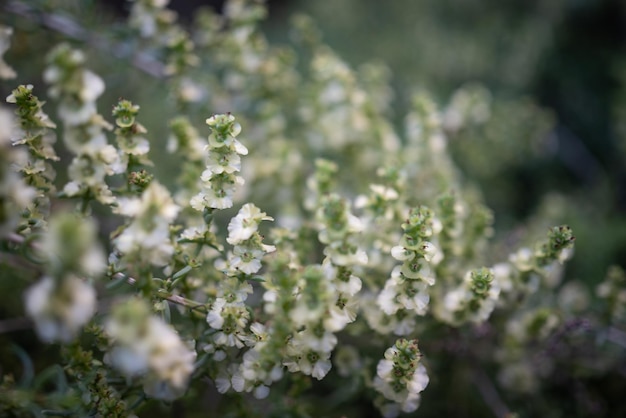This close-up photograph captures an abundance of small white flowers blooming on green stems, set against a blurry background that hints at a dense growth of similar plants. The main subject is a bush with numerous flower clusters, each with delicate white petals surrounding green buds, attached to brownish-green branches. While the precise number of flowers is indistinguishable, the image conveys a sense of profusion, possibly suggesting hundreds of blooms. The background, out of focus, contains additional flowers and greenery, creating an impression of an outdoor setting or perhaps a greenhouse. The image features some dark green foliage from a different plant on the right side and a hint of purple in the foreground, adding depth and contrast to the predominantly green and white composition.